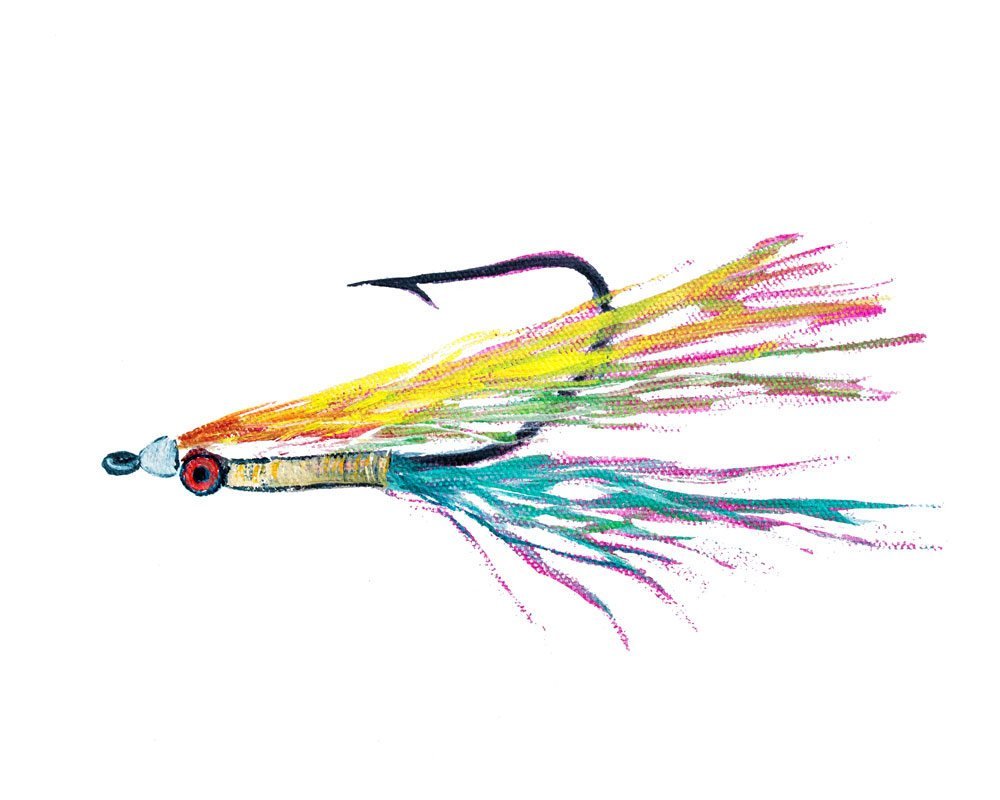This detailed illustration features a black fishhook lure drawn in pencil, lying horizontally against a white background. The hook itself, positioned centrally, curves to the left, with its sharp point directed upward and back towards the left. Radiating from the hook are an assortment of brightly colored feathers and threads in hues of red, yellow, green, pink, turquoise, and purple, designed to conceal the hook and attract fish. At the far left end of the hook, there's a small circular eyelet for attaching it to a fishing line. The meticulous details suggest a blend of mediums, potentially including pencil, crayon, or pastel, highlighting the artist’s craftsmanship in creating a vibrant and functional piece of fish tackle artwork.